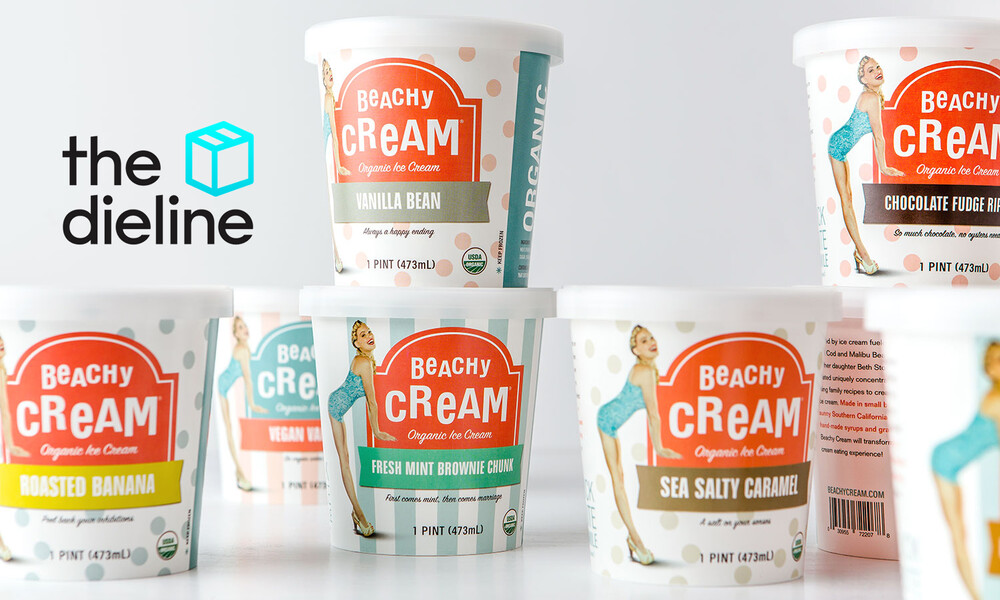This color photo advertisement for Beachy Cream ice cream features eight pints of the dessert displayed on a white tabletop in a seemingly random arrangement. Most pints have their retro-style logos facing the photographer, depicting a woman in a 1940s or 1950s bathing suit, evoking a vintage feel. The main logo, adorned with whimsical white font on a red background, reads "Beachy Cream" with "organic ice cream" italicized beneath. Despite its nostalgic aesthetic, the ad is distinctly contemporary, highlighted by the modern “dye line” logo with a turquoise cube in the upper left corner. Flavors on display include Vanilla Bean, Roasted Banana, Fresh Mint Brownie Chunk, and Sea Salty Caramel, emphasizing a blend of classic and inventive tastes. The pints feature both white and blue caps, adding a touch of variety to the presentation.